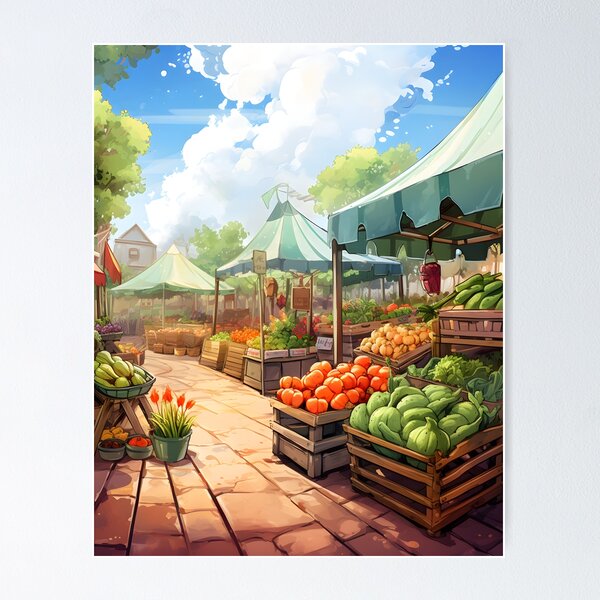The image is a detailed digital illustration of a bustling farmer's market. The scene is set under a series of large, striped canopies with alternating green and white or turquoise and dark turquoise patterns, giving off a vaguely medieval vibe. The market stalls are filled with a vibrant array of produce displayed in wooden crates. In the foreground, prominent crates showcase green leafy vegetables and various types of squash in hues of green, orange, and butternut. Further into the image, other colorful vegetables including red and purple varieties can be seen, though they are less distinct. 

A metal holder on the left displays a bouquet of red tulips, adding a splash of color to the otherwise earthy tones. Adjacent to this, on the ground, lies a stone pathway of orange and light brown bricks that leads off to the left side of the image. Flanking the pathway are green trees, and in the background, a white building with a pointed roof stands under a bright blue sky filled with scattered white clouds. The overall atmosphere is lively and sunlit, capturing the essence of a vibrant, sunny day at a traditional farmer's market.